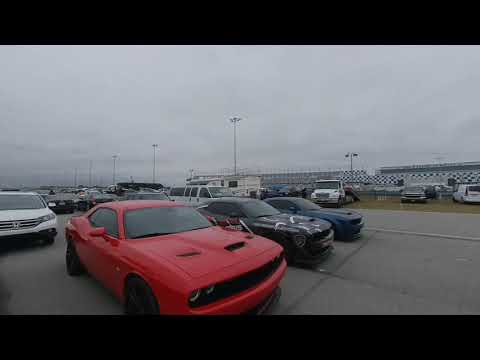The image displays a parking lot adjacent to a racetrack under a distinctly gray, cloudy sky. In the foreground, several sports cars are parked diagonally. Prominently featured is a custom red Camaro—possibly a newer model—flanked by a black sports car with white stripes and a blue one with black accents, which could be Dodge Challengers. The scene includes various other vehicles like vans, sedans, SUVs, trucks, and a motorhome, all arranged neatly in the background. The racetrack setting is suggested by the checkerboard pattern along the structures and several tall light poles scattered around. The image is bordered at the top and bottom by black, emphasizing the central placement of the vehicles, while the surrounding area hints at stands and further asphalt pavement. The overall ambiance is muted due to the overcast conditions, casting a grayish tint over the entire scene.